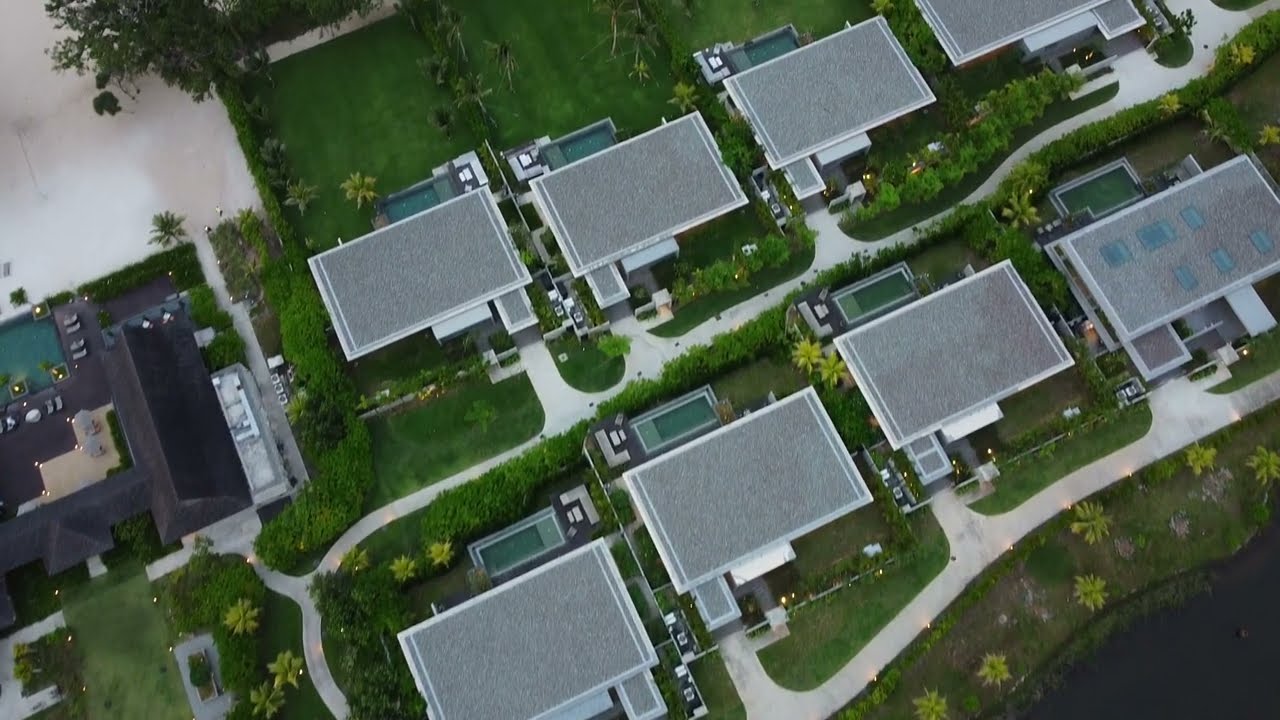This aerial photograph, taken from an aircraft or drone at an altitude of approximately two to three hundred feet, offers a detailed top-down view of a uniform neighborhood, likely a retirement community. Dominating the left side of the image is a larger building, possibly a clubhouse, surrounded by green lawns, bushes, and palm trees. This building is bordered to the upper left by a white paved area, likely a parking lot. The clubhouse features a larger backyard with walkways connecting to other parts of the community.

The neighborhood's main section comprises multiple rectangular, modern-looking houses with flat gravel roofs. Each house has a small backyard, often featuring tiny lap or swing pools, separated by hedges. The backyards also contain manicured lawns and garden pathways interlinking the houses, creating a cohesive, well-maintained appearance. In the lower right of the image, there is a dark-colored body of water, further emphasizing the serene environment of the locale. The abundance of greenery, uniform landscaping, and the presence of pathways underscore the area’s organized and tranquil nature.